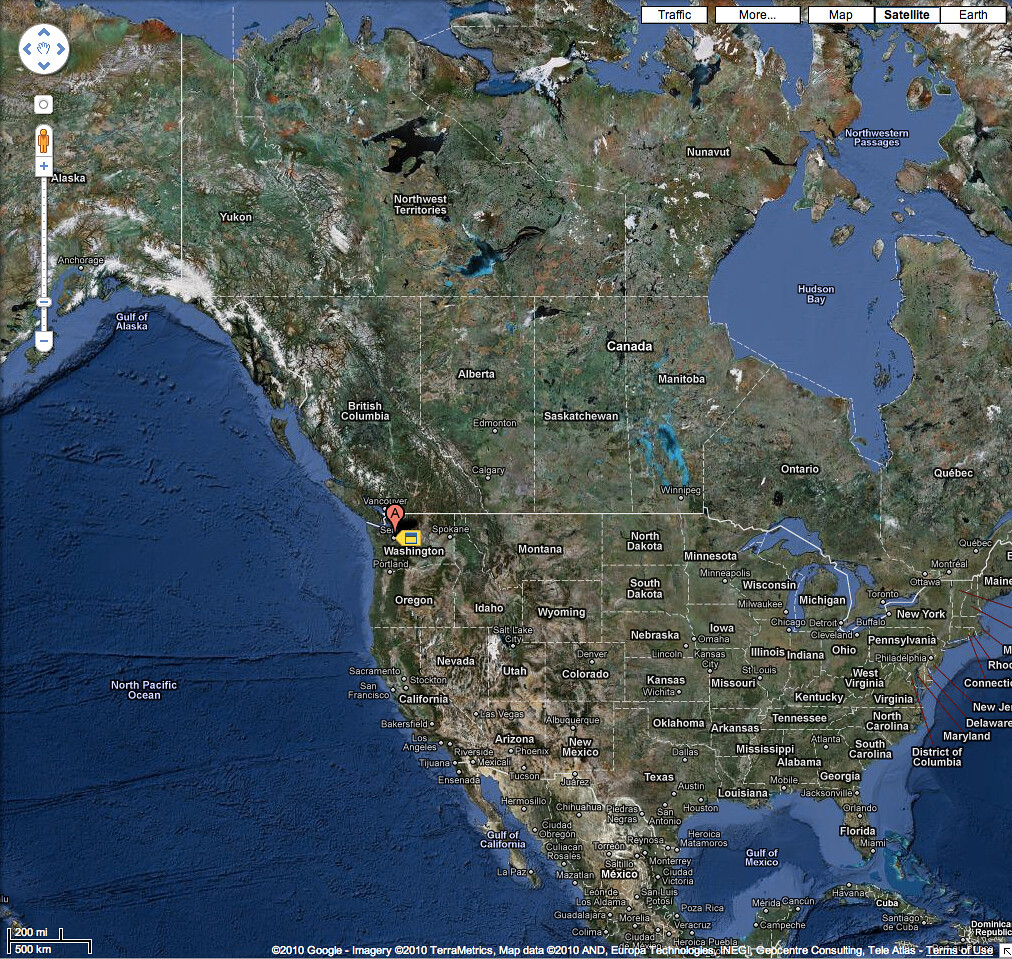This is a detailed satellite image from Google Maps depicting North America. The map features a full view from the northern regions, including the Yukon, the Northwest Territories, and Hudson Bay, down to the southern regions showcasing Mexico, the Gulf of Mexico, and the Caribbean islands of Cuba and the Dominican Republic. The left side illustrates the expanse of the North Pacific Ocean, while the east coast highlights states like Maine, New York, and Florida. Landmark bodies of water such as Hudson Bay and the Gulf of Mexico are clearly labeled. Geographical details like the mountain ranges, prairie lands, and the white peaks of the Rocky Mountains are vividly depicted. The map includes provincial boundaries in Canada, state boundaries in the United States, and distinguishing labels for regions and bodies of water. At the bottom, there are notations including "2010 Google Imagery, Terrametrics," along with a distance scale. Overlapping features from different descriptions provide a comprehensive and clear view of the North American continent on Google Maps.